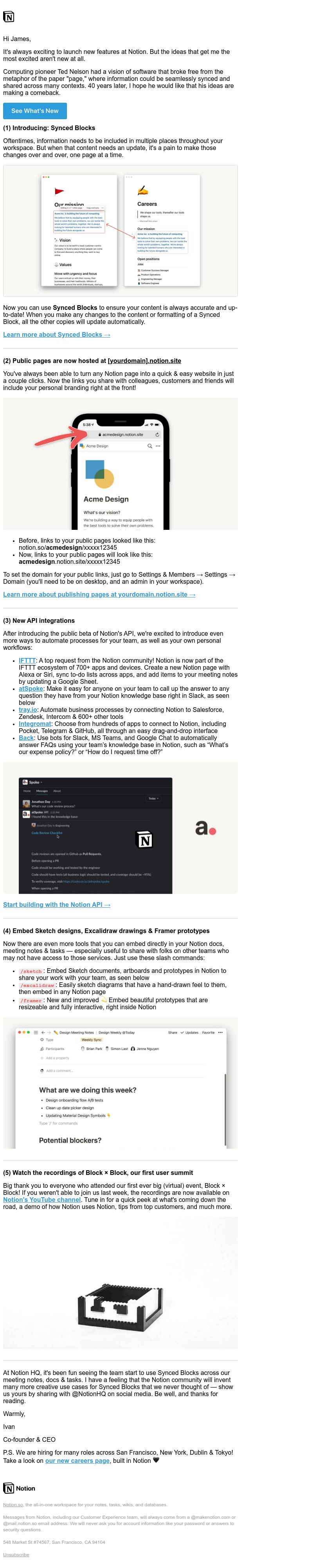The image displays a densely textual document with various formatting elements that are difficult to decipher. On the left-hand side, a flashing vertical black line grabs immediate attention, alternating between on and off states. The document comprises multiple lines of text interspersed with a thick blue line, punctuated by a picture showing two separate pages. Despite the blurred legibility, some text appears at the beginning of certain lines in blue lettering, adding to the visual complexity. Intermixed within the text is a distinctive black script featuring a lowercase "a." The overall scene suggests a highly formatted page with significant visual segmentation and highlighted sections.